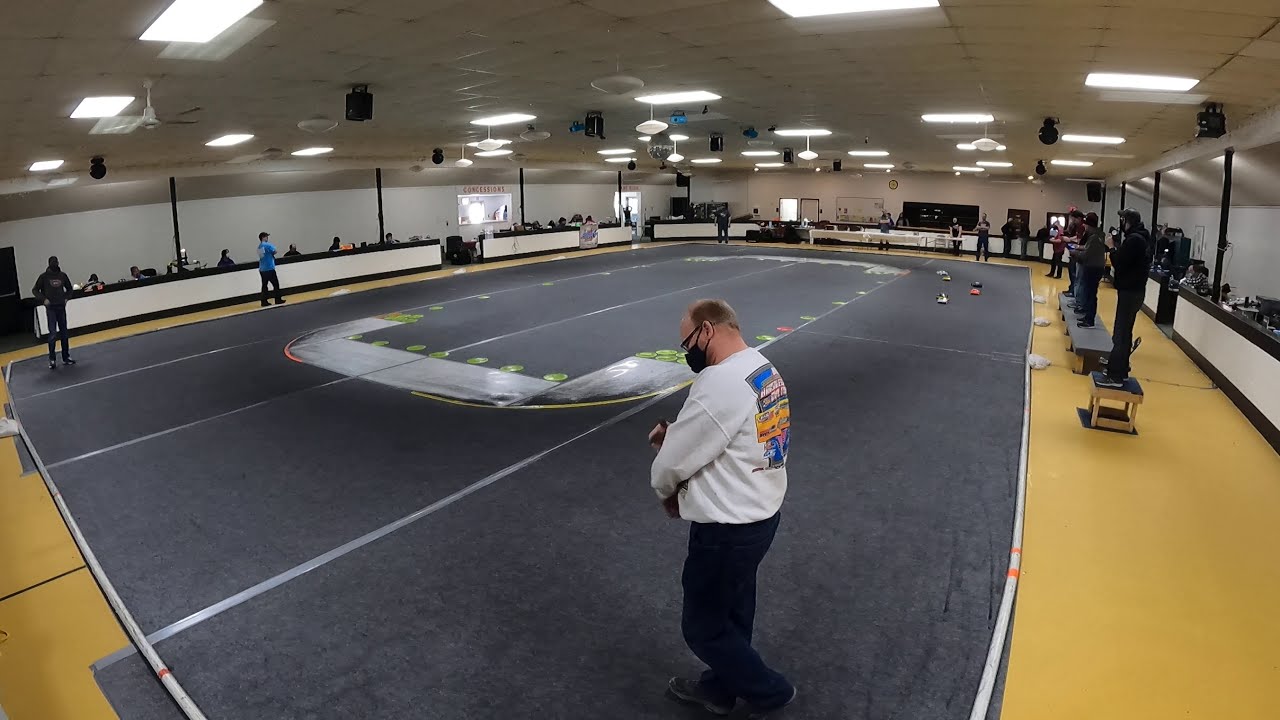The image depicts an indoor arena, resembling a gymnasium with low, tiled ceilings adorned with bright fluorescent lights and spotlights. The large, horizontally aligned rectangular room has yellow-bordered brown tile flooring surrounding a substantial dark gray area with white and light gray stripes, possibly functioning as an RC (remote control) car track. The grayscale track is outlined in an oval shape, marked by white lines and tape for guidance. In the foreground, a man is seen standing on the track, wearing a long-sleeve white shirt with graphics on the back, black pants, boots, eyeglasses, and a black mask, focused downward, suggesting engagement with the activity. Along the right side of the image, several individuals stand on stools, holding remote controllers, likely operating the small RC cars visible on the track. Additional people are gathered on benches and behind a low white panel that separates the track from the spectator area, contributing to the bustling atmosphere of the room. The background is characterized by white walls and more seated spectators, adding to the organized yet vibrant setting. The overall ambiance is brightly illuminated, showcasing a well-lit and expansive indoor recreational space.